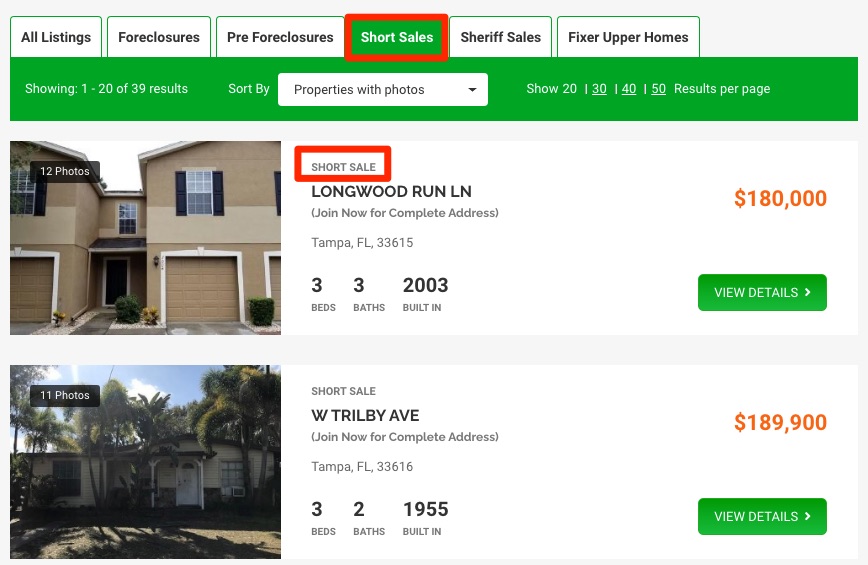This screenshot showcases a computer monitor displaying a real estate platform focused on various property listings. The top of the screen features multiple tabs labeled "Listings," "Foreclosures," "Pre-foreclosures," "Short Sales," "Sheriff Sales," and "Fixer-Upper Homes." Just below these tabs, a green section indicates, "Showing 1 of 20 of 39 results," alongside a sortable dropdown menu labeled "Properties with Photos." To the right, there is an option to display either 20, 30, 40, or 50 results per page. 

The main content of the screen displays images of two featured properties. The first property is marked as a short sale. It is a tan, single-family home featuring a front view with a two-car garage, private entrance, some surrounding brush, and a driveway. The listing states that the home is located on Longwood Run Lane in Tampa, Florida, ZIP code 33615. It offers three bedrooms and three bathrooms, was built in 2003, and is priced at $180,000. There is a green "View Details" button available for more information.

The second property, also under a short sale, is depicted under sunny skies with palm trees. It appears to be a one-level home with 11 photos available. The property is located on W. Tripoli Avenue in Tampa, Florida, ZIP code 33616. It includes three bedrooms and two bathrooms, was built in 1955, and is listed at $189,900. Like the previous listing, it features a green "View Details" button for additional information.